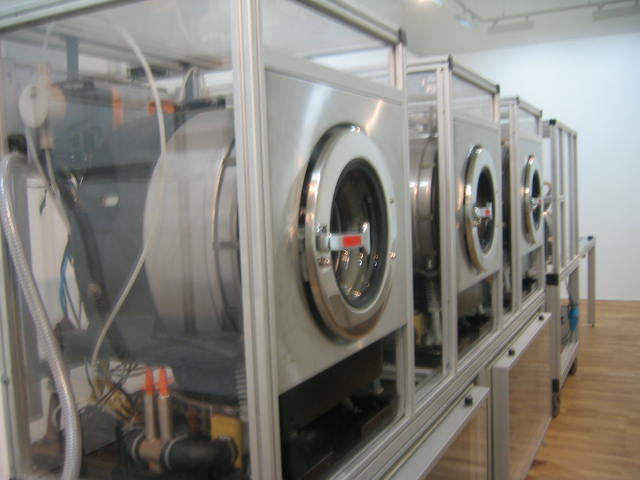In this color photograph, we're looking at what appears to be a row of pristine commercial laundry equipment that could either be front-loading washers or dryers. These stainless steel units, with their circular glass doors and silver levers, are lined up diagonally from the left side of the image extending back into the depth of the frame almost reaching the right side. Each unit stands elevated on a platform, showcasing their legs and the intricate machinery on the sides, consisting of exposed dark grey and light grey metals interspersed with red and yellow wiring. The backdrop features a clean, white wall and the floor is a polished, variegated brown wood, an unusual but elegant choice for such an industrial setting. The ceiling hosts industrial lighting, and the exposed piping finishes with a touch of orange at the tips, matching the small orange accents found on the equipment handles. Overall, this visually striking scene is likely a display setting, showcasing these machines in an environment that blends industrial robustness with refined aesthetics.